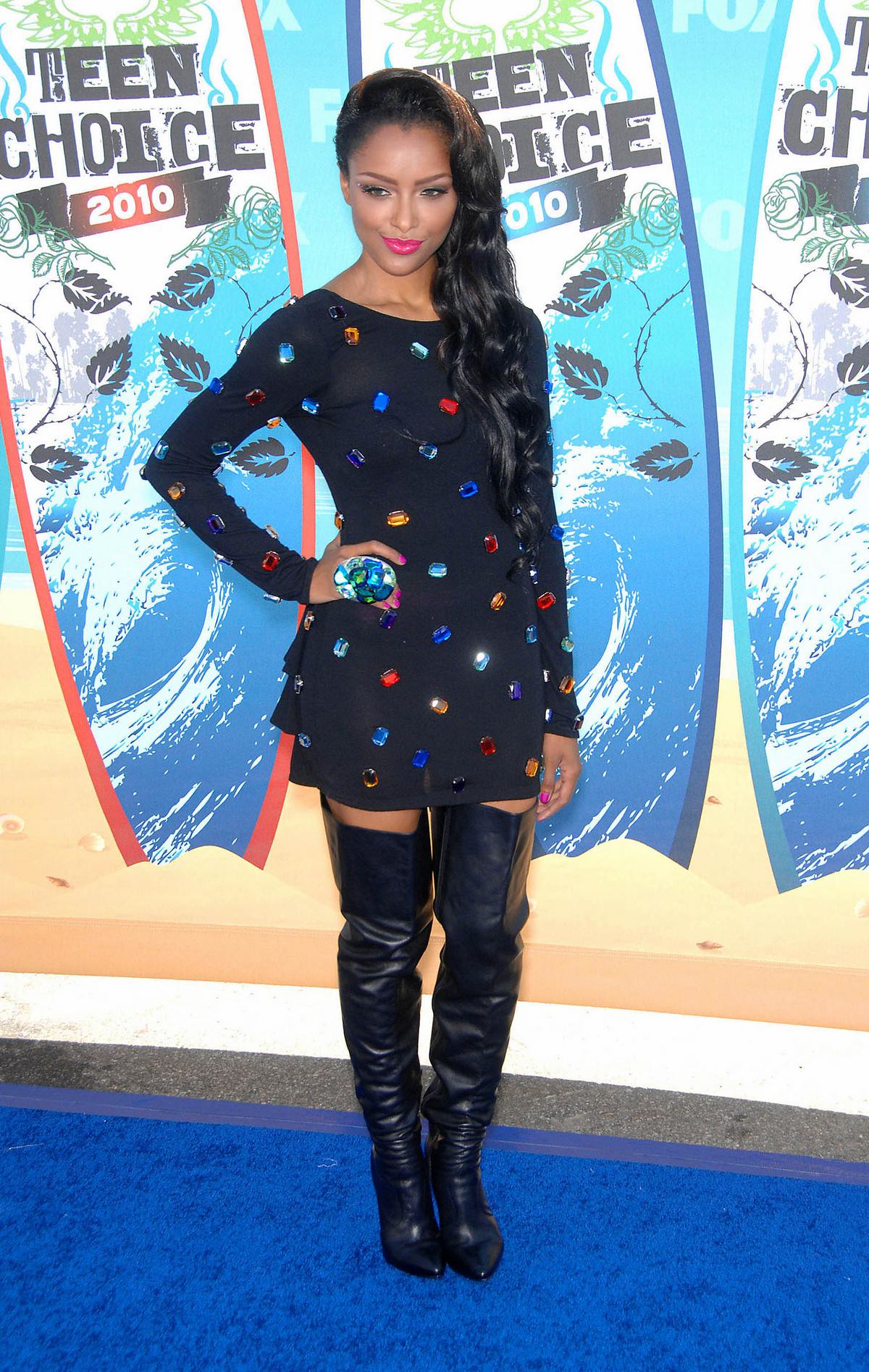The image features a slightly dark-skinned woman, possibly an actress or model, posing on a blue carpet in front of a display that reads "Teen Choice 2010." The background includes surfboard-like symbols adorned with waves, leaves, and gray lettering. The woman has long, flowing black hair swept over her left shoulder down to her waist, and she is wearing pinkish-red lipstick. Her outfit comprises a long-sleeved, somewhat sheer black dress adorned with small gemstones in blue, red, and white, creating a sparkling effect. The dress extends to her upper thigh, just above her thigh-high black leather high-heel boots, leaving a small section of her bare thighs visible. She has pink nail polish and a large, gem-studded ring covering several fingers on her right hand, which is resting on her hip. Her left arm hangs by her side. She projects a confident, smoldering look with a closed-mouth smile as she poses for the camera.